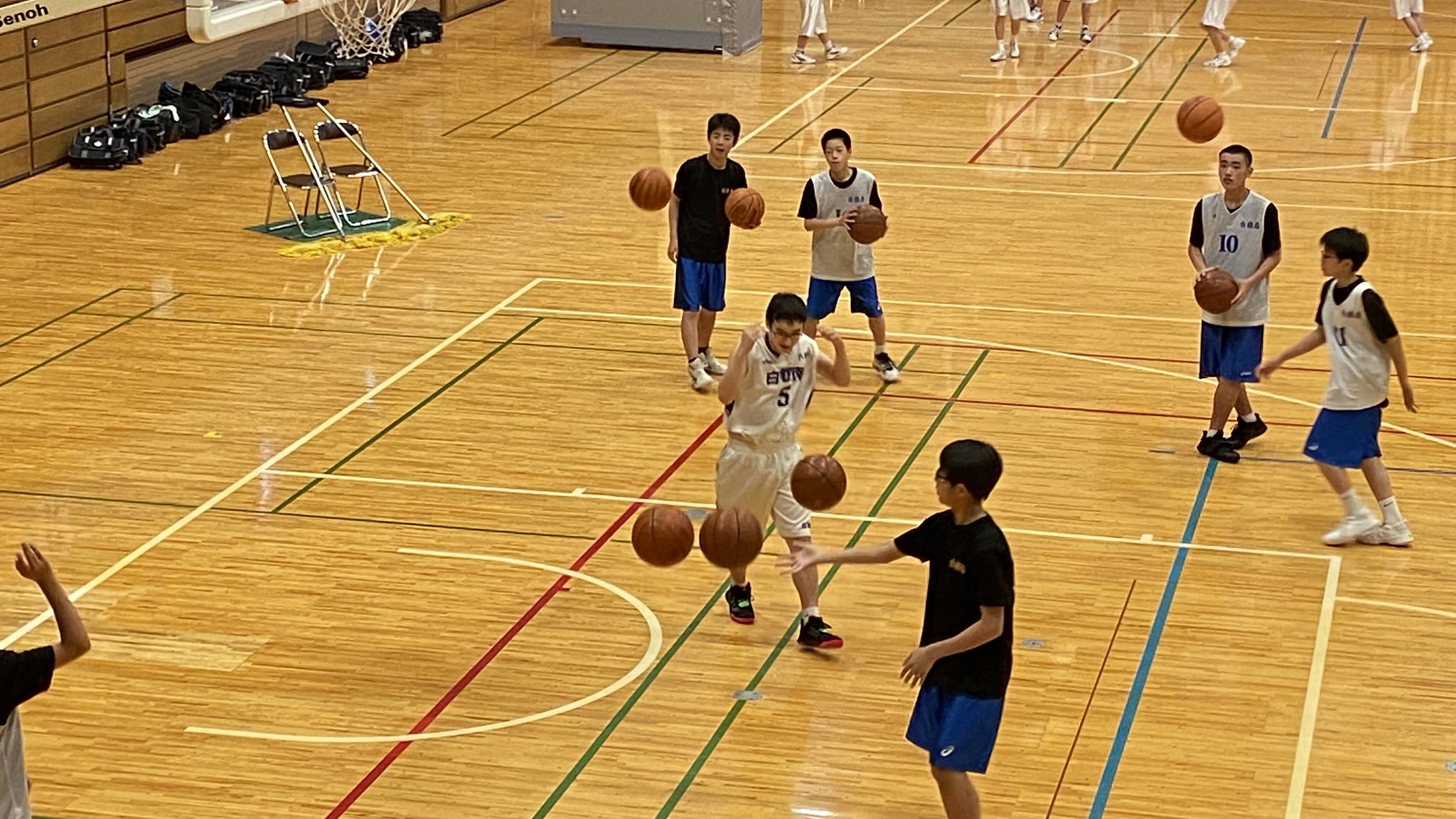In this vibrant and dynamic photo taken inside a high-gloss, indoor basketball gymnasium, a group of young Asian men, likely high school students around 15 years old, are actively engaged in various basketball drills on a marked court. Most are donned in white jerseys paired with dark blue shorts, while two sport black t-shirts with matching dark blue shorts. The floor is characterized by its shiny finish, adorned with a spectrum of basketball markings in red, blue, and green.

Approximately eight young men are prominently visible on this section of the court, with at least three basketballs captured mid-air, emphasizing the intensity and simultaneous nature of their drills. Some players are wearing glasses, adding a personalized touch to their athletic attire. In the midst of practice, one young man is poised with a ball in his left hand, another grips a ball with both hands, seemingly ready for action, while a third, positioned on the side, appears to be preparing to shoot.

In the background, the legs of additional players in white shorts can be seen, implying the presence of another team. The scene is further enriched by the sight of gym bags lined along the back wall and a basketball net hanging from the left side of the frame. The overall context suggests a bustling environment filled with energetic, coordinated activity, capturing the essence of youth sports and teamwork.